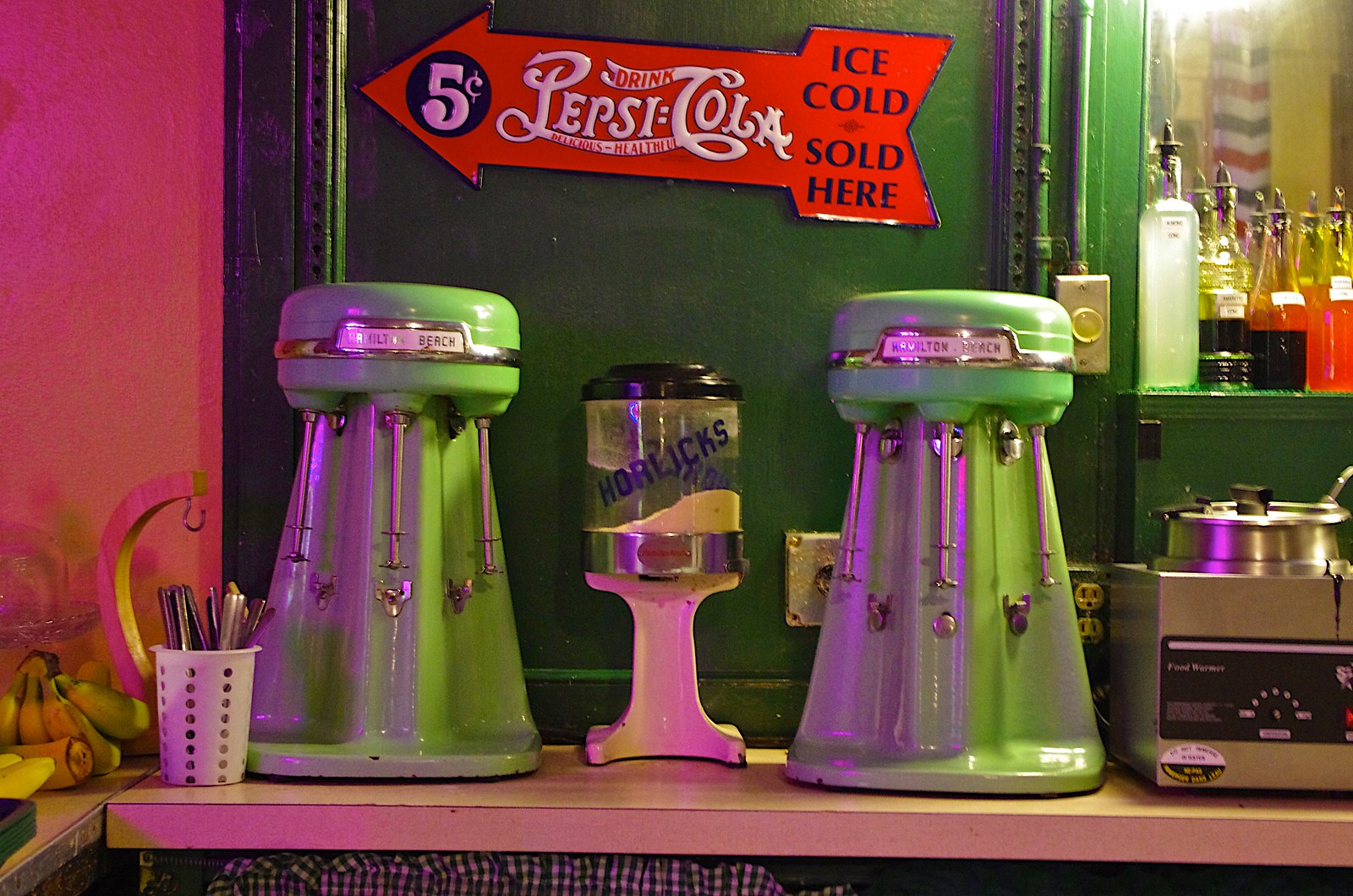The image features a vibrant preparation counter in a diner or bar with various kitchen equipment and accessories. Dominating the scene are two identical green machines, likely blenders or mixers, positioned on the left and right sides of a white wooden counter. Each machine is equipped with three metal sticks topped with round cups and conical lower sections, suggesting they are used for making milkshakes or similar beverages. Between them, there is a glass container labeled "Horlicks" on a white stand, containing a yellow powder. Above the counter, a retro red arrow sign reads "Pepsi Cola, Ice Cold, Sold Here, 5 cents," set against a green wall. The counter also features a white circular container holding utensils, situated near a bunch of green bananas and a wooden banana stand. Additionally, to the right, there are various bottles, possibly containing syrups or flavors, and a warming stove with a handle, potentially for serving hot fudge. The far left of the image has a background with a red, rose-colored wall.